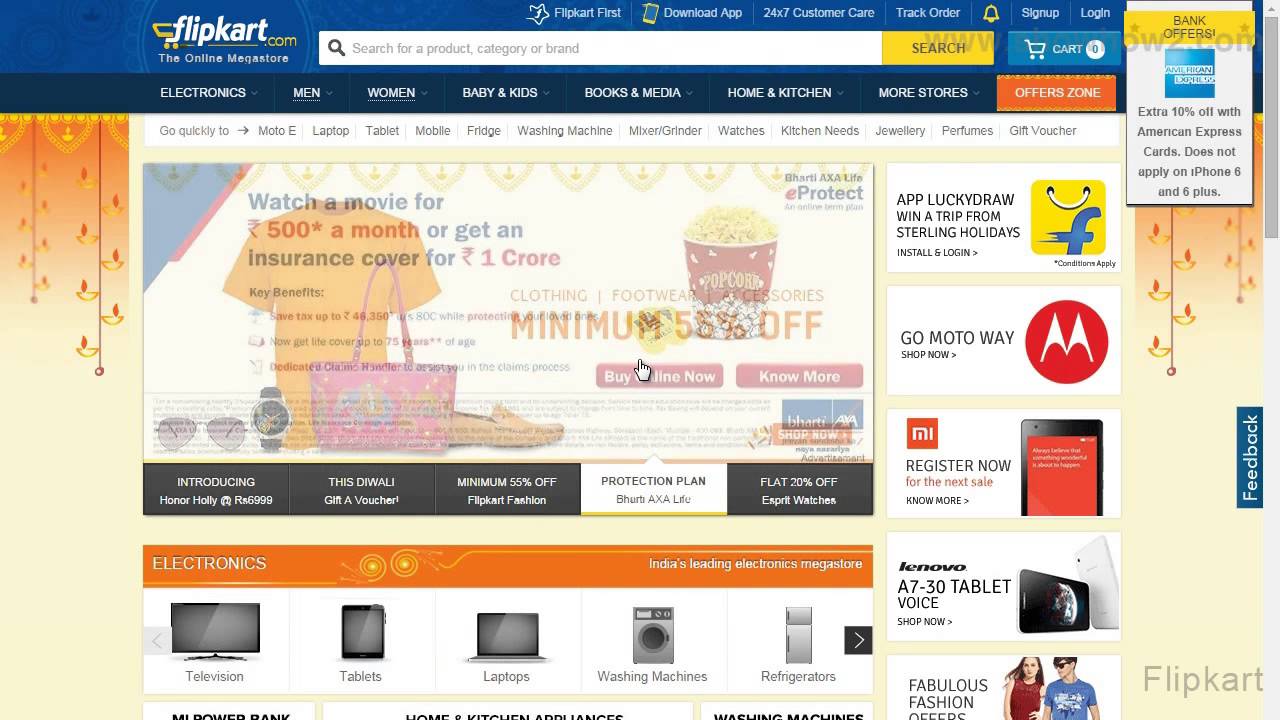This image captures the homepage of the Flipkart website. The top border, about an inch down, is shaded in medium blue. Approximately two inches from the left side, the word "Flipkart" appears in white text, accompanied by the subtitle "the online megastore" also in white. Adjacent to the "Flipkart" logo, there's a yellow ".com". Dominating the central part of the webpage is a large white search bar, which spans about half the width of the image. Next to the search bar, a yellow tab with the word "Search" in blue is visible. 

To the right of the search bar, there's a light blue tab featuring a white cart icon and the word "Cart" in white. In the upper right corner of the page, a white circle encloses a dropdown tab, topped with a yellow banner that reads "Bank Offers" in black text. Below this banner, there's an American Express icon with additional related information.

Above the search bar, there are six different dropdown tabs, including options for "Login" and "Sign Up". Further below these options, a dark blue tab houses six more dropdown tags in white, listing categories such as Men, Women, Kids, Books, and Media.

On the left side of the page, there is a section with a dark orange top that fades into a lighter orange as it descends, bordered by a yellow line at the top. Between these borders, the background is entirely white. A large square in this section provides details about a shopping offer: "Watching a movie for $500 a month." To the right of this square, there are five clickable rectangles offering various options.

Beneath this, on the left side, an electronic section with an orange border displays the word "Electronics" in white text. Under this heading, icons for different electronic devices such as a television, tablet, laptop, washing machine, and refrigerator are neatly arranged.